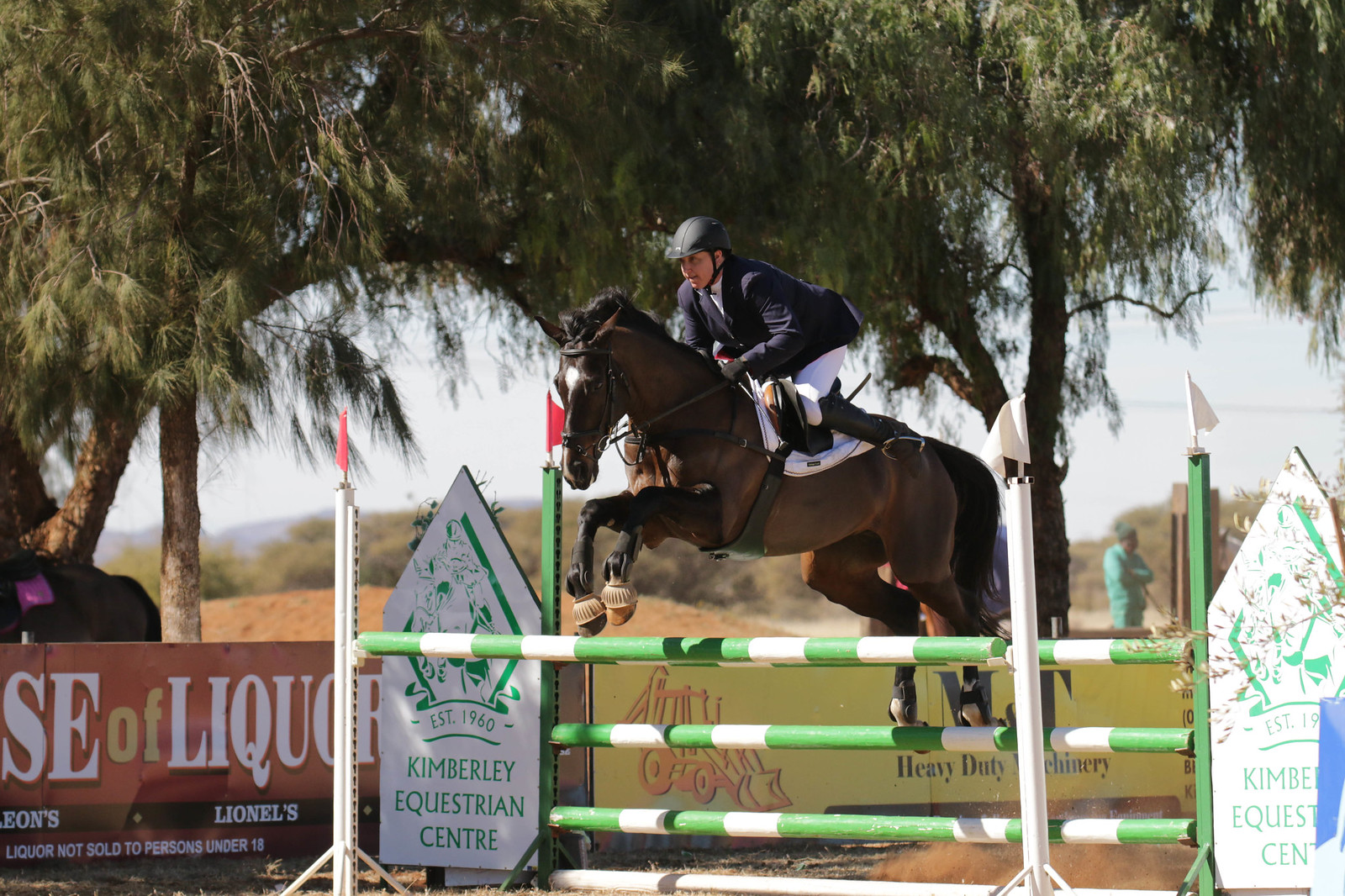In this vibrant image taken on a sunny day, a dark brown horse with black mane is captured mid-jump over a green and white striped fence. The rider, donning a blue helmet, a navy jacket, and white pants with riding boots, adeptly guides the horse through the air. The scene is set against a backdrop of lush greenery and a large dark green tree with drooping leaves. Various advertisements for heavy-duty machinery, a liquor company, and the Kimberly Equestrian Center EST 1960 are visible. The sky is a clear, haze-tinted blue, adding to the picturesque setting of the equestrian event.